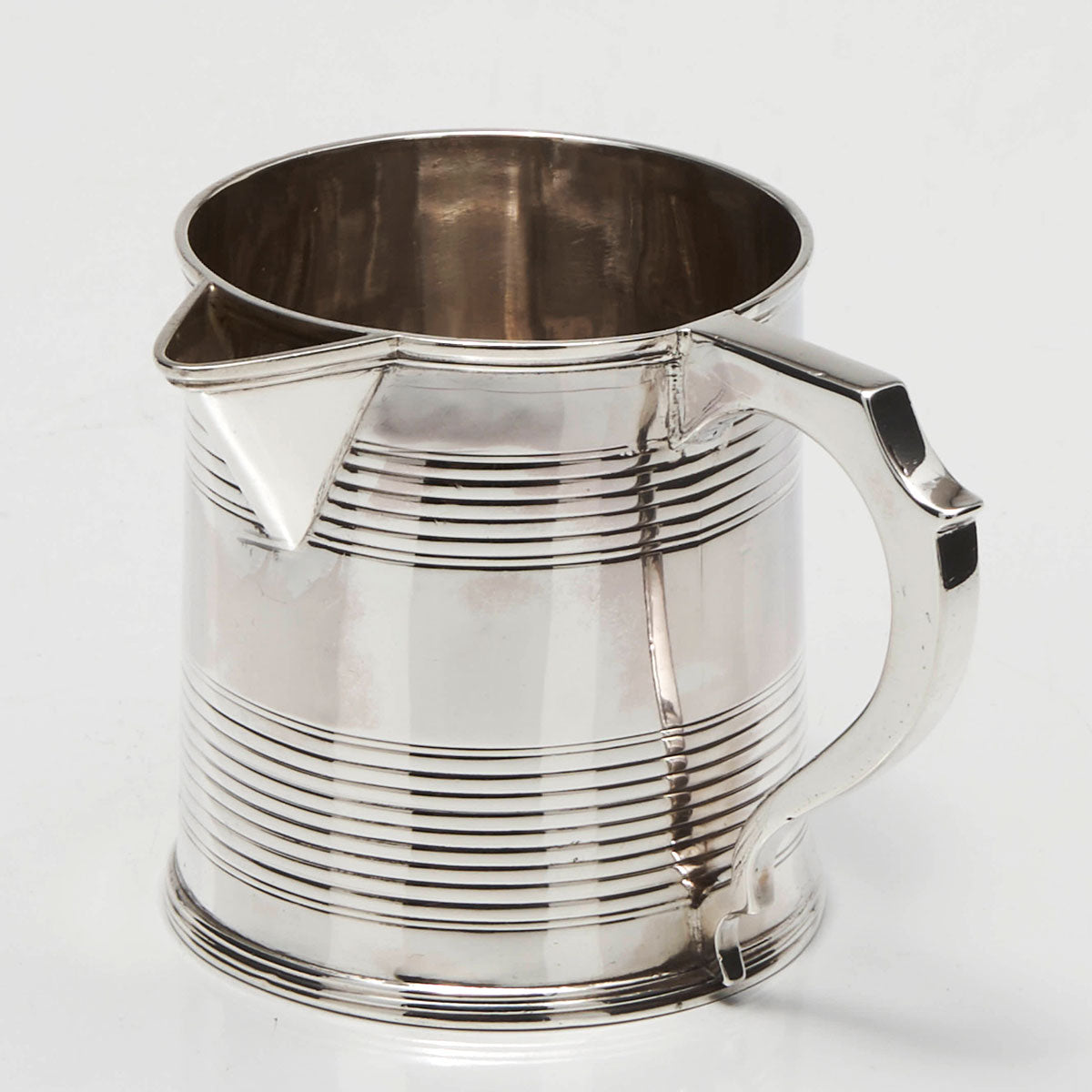This close-up image features a highly reflective stainless steel pitcher with a sleek design, resembling that of a cup or mug. Positioned on the right side, a sturdy handle seamlessly integrates into the body of the pitcher, which is currently empty, revealing a hollow internal cavity through its open top. The top-left rim showcases an outward-jutting spout designed for pouring. Delicate fine lines, visible across the surface, run horizontally along the top and bottom portions of the pitcher, adding texture to its smooth, chrome-like sheen. The entire composition is set against a stark white background, accentuating the pitcher’s polished, mirror-like finish.